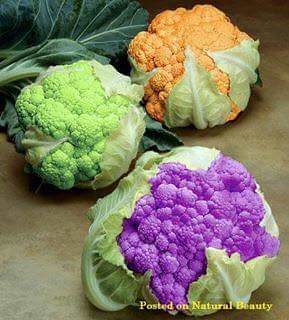This vertically-oriented color photograph features a remarkable display of three distinct heads of cauliflower, each uniquely colored. Dominating the upper left corner is a large, deep green cauliflower leaf, adding a lush touch to the composition. To its right, one cauliflower head, adorned with bright orange florets, faces the camera. Flanking this orange cauliflower on the left, another head showcases light green florets. In the foreground, a third cauliflower head proudly exhibits its vivid violet-purple florets. All three heads are neatly arranged on a diffused, brownish-gray table, providing a neutral yet complementary backdrop. The image, which appears to be captured with a higher-quality camera and possibly digitally enhanced, also features a bottom watermark reading, "Posted on Natural Beauty."